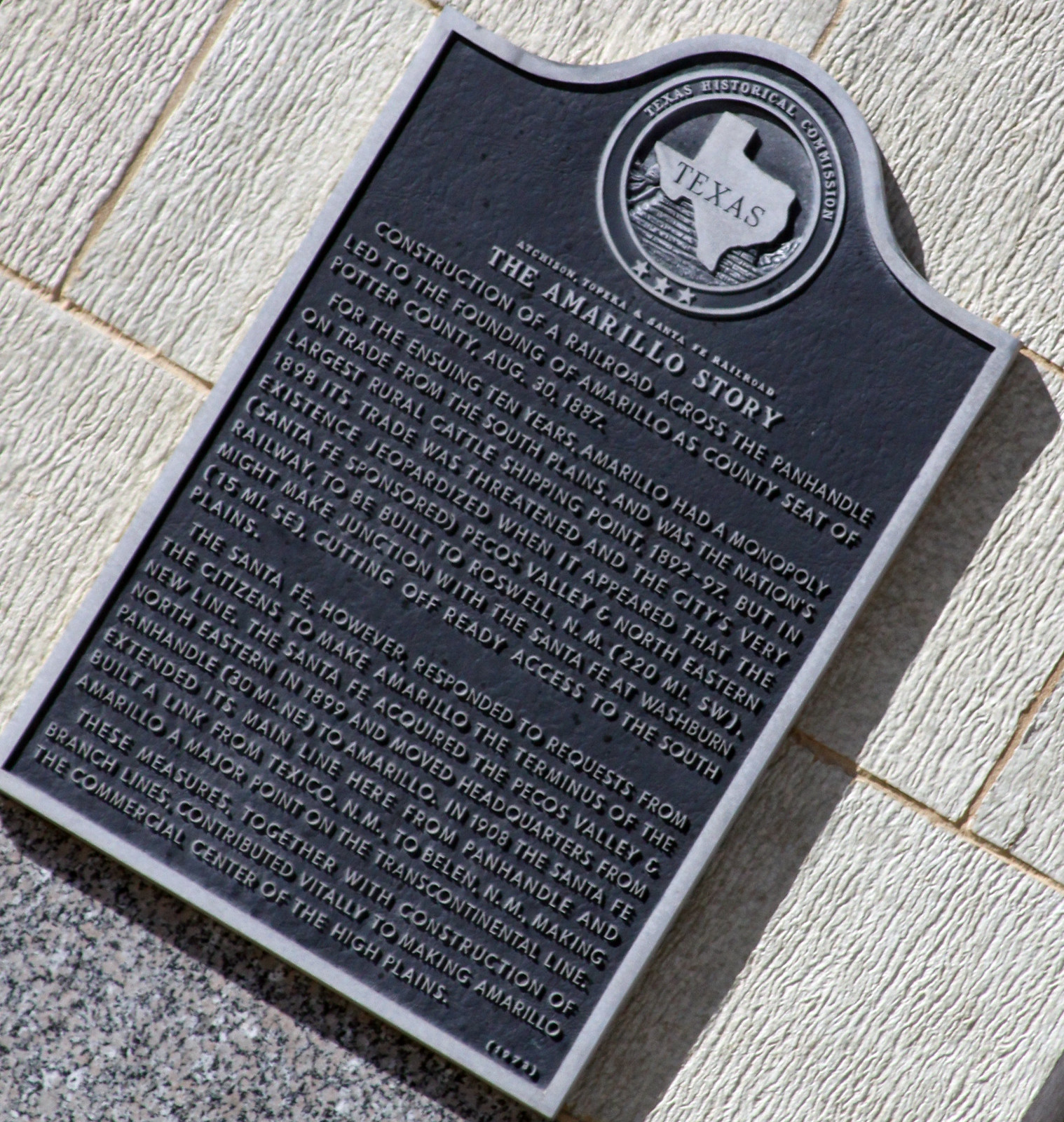The image captures a detailed photograph of a historical marker affixed to a large, roughly textured white stone wall. The rectangular plaque, positioned diagonally with its top pointing towards the top right corner of the frame, is crafted from metal and features a striking design. It has a silver-gray border framing a black background with white raised letters. At the very top of the plaque is a circular emblem bearing the Texas Historical Commission's name, encircling an outline of the state of Texas with the word "Texas" inscribed within.

Beneath this emblem, the raised text begins with "Atchison, Topeka, and Santa Fe Railroad, the Amarillo story." The plaque narrates the history of Amarillo, focusing on the pivotal role played by the construction of a railroad across the Panhandle. This development led to Amarillo being designated as the county seat of Potter County on August 30, 1887. From 1892 to 1897, the city held a monopoly on trade from the South Plains and was recognized as the nation's largest rural cattle shipping point. However, in 1898, Amarillo's trade dominance and existence were threatened when the Santa Fe-sponsored Pecos Valley and Northeastern Railway planned a route that might bypass the city. The Santa Fe Railroad, responding to citizens' requests, decided to make Amarillo the terminus of the new line. By acquiring the Pecos Valley and Northeastern in 1899 and relocating its headquarters to Amarillo, along with extending its main line and adding new links, Amarillo emerged as a major hub on the transcontinental railway. These developments solidified Amarillo's status as the commercial center of the High Plains, significantly contributing to its growth and prominence.